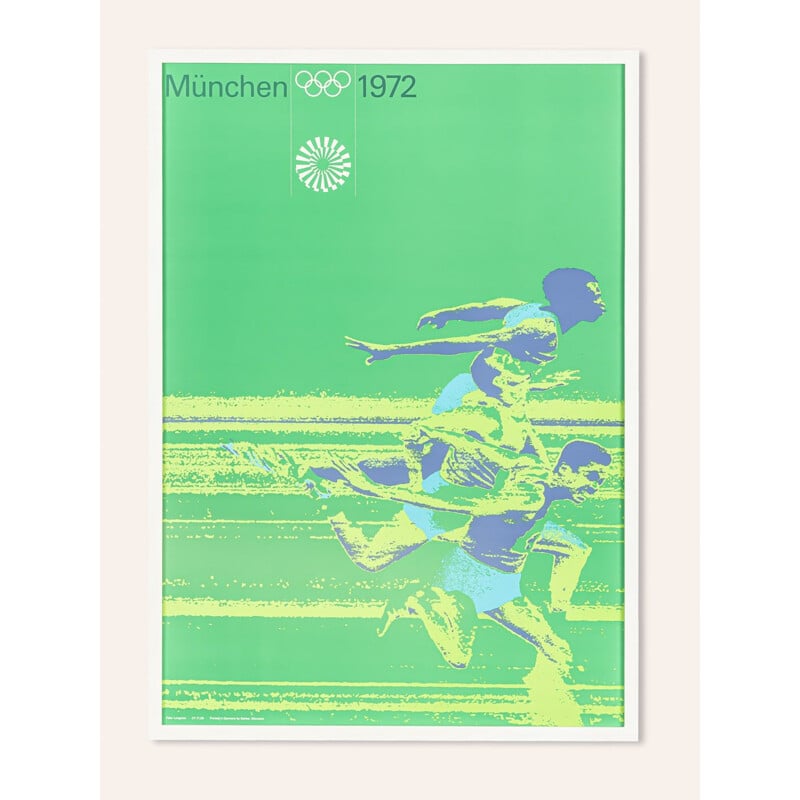This framed artwork, likely a poster from the 1972 Munich Olympics, features a distinctive design with a light green background and is enclosed in a white frame. At the top left corner, the poster prominently displays the text "München 1972" and the iconic five Olympic rings in white. Directly beneath the rings is a white circular symbol, which resembles a sun. The main image depicts an animated and sketch-like scene of three runners sprinting to the right, each characterized by unique physical traits and clothing. The top runner appears to be Black, the middle runner is probably White, and the bottom runner might be Hispanic. All three athletes are dressed in light blue shorts and purplish tops, with some areas of their skin tinted purple. Light yellow horizontal lines streak across the lower portion of the image, adding to the dynamic feel of the runners racing, seemingly towards a finish line.